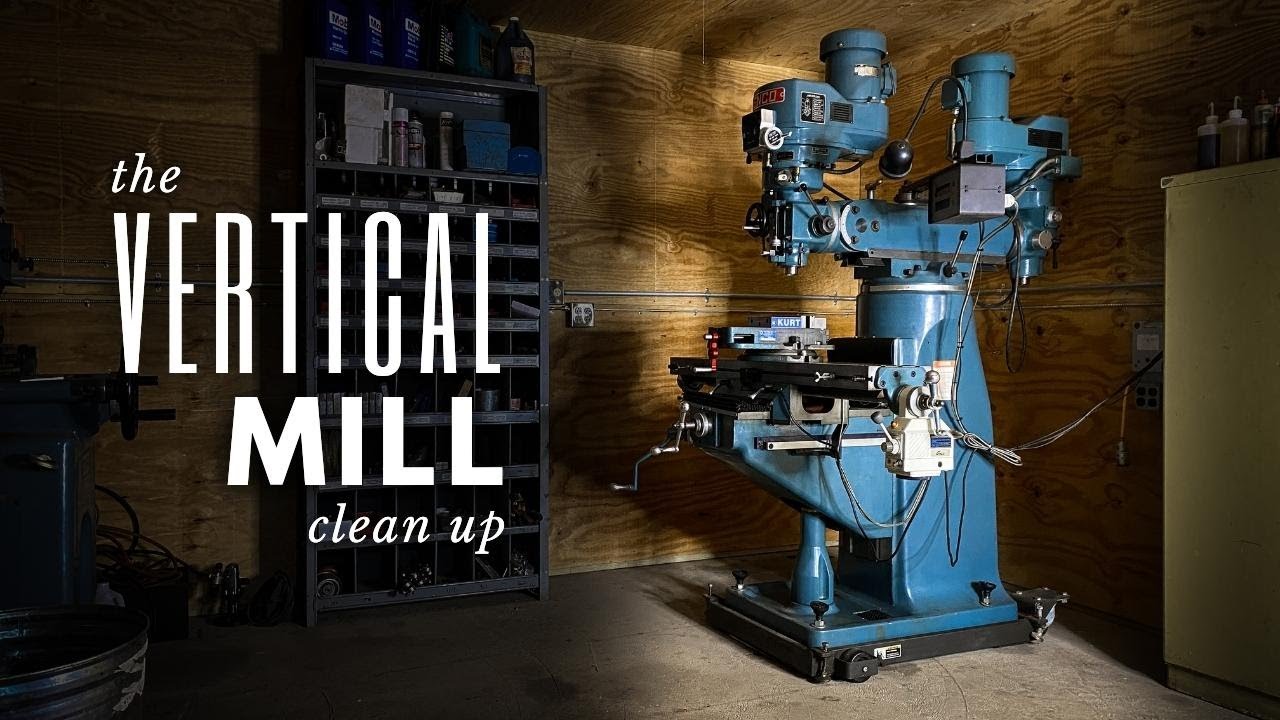The image depicts a complex, mobile mechanical device, likely used for manufacturing or machining, featured prominently in a workshop with light brown plywood walls and a gray cement floor. The blue-colored machine, which appears to be a vertical mill, is equipped with numerous wires and various compartments. It is positioned on the right side of the room near the wall, illuminated by focused lighting, and placed on a set of wheels, indicating its mobility. This machine has an area resembling a clamp for securing materials and a stamper-like component above. Electrical wiring runs throughout the room, with outlets spaced regularly. To the left of the machine, there is an old refrigerator with bottles on top, and a metal shelf housing various tools and brackets. The left side of the image contains white italic and capitalized text that reads "the vertical mill cleanup." The surrounding storage units and workshop details hint at a functional and well-used space, likely dedicated to woodworking or similar activities.